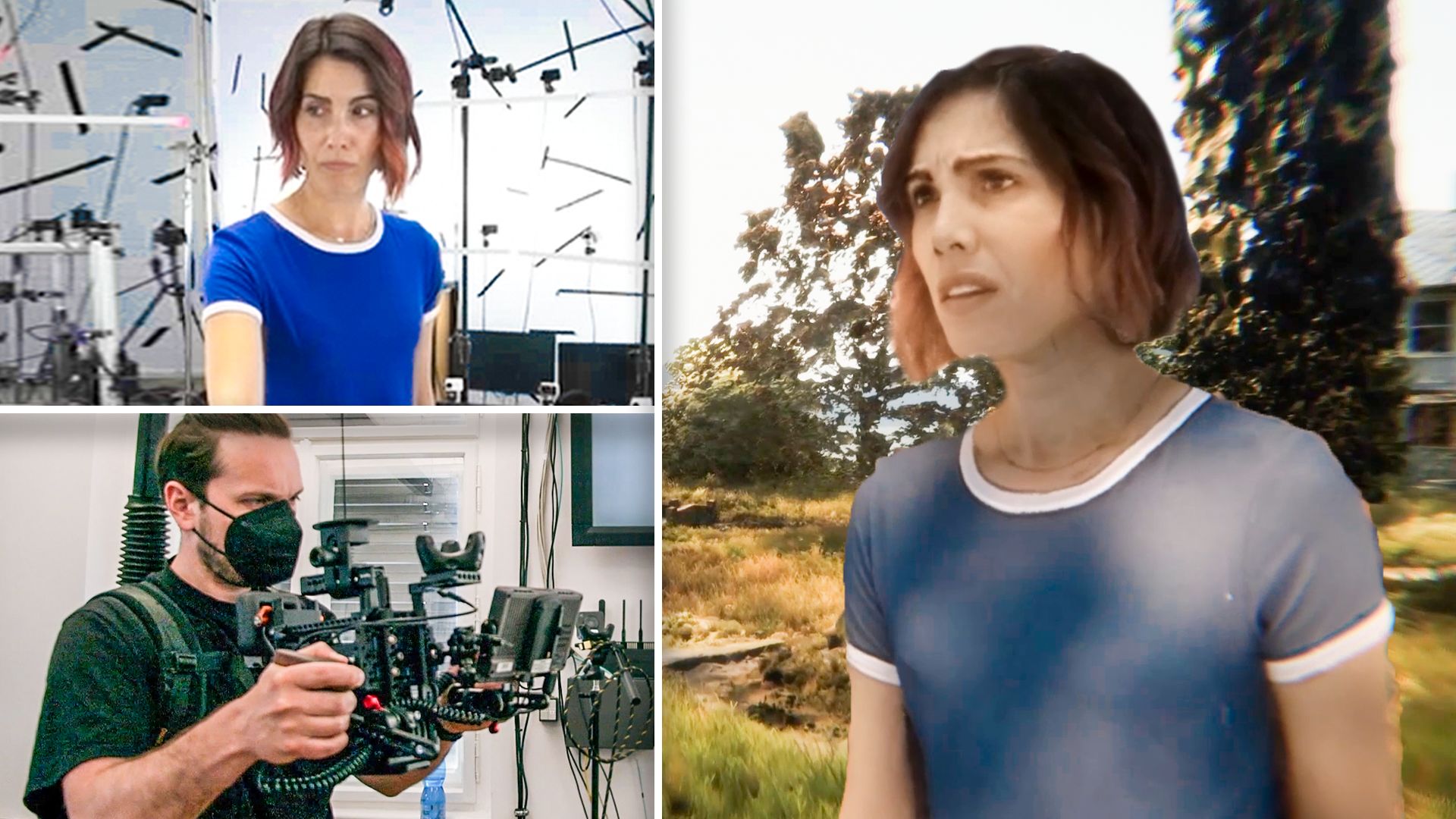The image is divided into three distinct sections, with one larger section on the right and two smaller sections on the left. In the larger, right-hand section, a brunette woman with shoulder-length hair stands outside, wearing a blue top with white detailing around the collar and sleeves. She is positioned in front of a backdrop that includes a building partially visible through lush foliage and grass, with a tree trunk also in sight.

The left side of the image is split into two smaller sections. The top left section features the same woman, now in an indoor setting that resembles a high-tech studio or recording facility. Despite the indistinct background, the blue top with white detailing she's wearing remains consistent. Floating camera components or technical equipment hover around her, suggesting an environment dedicated to media production.

The bottom left section portrays a man operating advanced camera equipment, indicative of a professional filming scene. He is dressed in a dark t-shirt and a black face mask, with short brown hair and a beard. His gear appears highly sophisticated, emphasizing the technical aspect of the shoot.

Overall, the image captures a behind-the-scenes glimpse of a media production, showcasing both on-set and studio environments. The woman’s striking appearance and consistent attire juxtaposed with the professional cameraman's detailed setup highlights the meticulous effort involved in capturing both outdoor and indoor scenes.